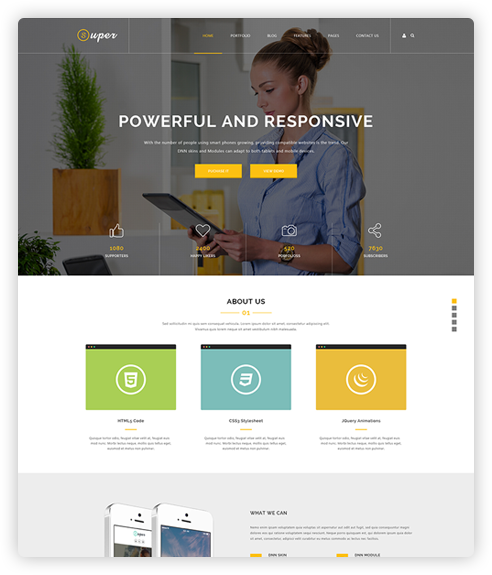The image depicts a website homepage with various elements. At the top-left corner, there's a logo featuring a yellow "S" inside a yellow circle, with the clear background behind letter. To the right of the logo, the word "UPER" is displayed in white text. The navigation menu located in the middle-right section includes links labeled "Home," "Portfolio," "Blog," and "Contact Us," although the menu labels are not entirely clear due to the poor resolution. To the far right are icons for user profile and search functionalities.

The background of the page features a photograph of a woman with brown hair tied in a bun, wearing a blue shirt, and looking at a tablet. She is positioned in a home-like environment with white walls and a green plant in a brown container visible. 

Overlaid on the background image are the words "Powerful and Responsive" in prominent white text. Below this, two lines of white text and two yellow buttons contain unreadable font due to the image's resolution. 

At the bottom of the page, there are icons for thumbs up, a heart, a camera, and a share button, with some additional unreadable text below them. Further down is a section titled "About Us" followed by what appears to be "01". 

Additionally, there are three circular indicators labeled "123" for navigating website pages, colored green, turquoise, and orange respectively. The green one includes partially readable text starting with "With". The area around this section has a white background, and all text within this section is unreadable.